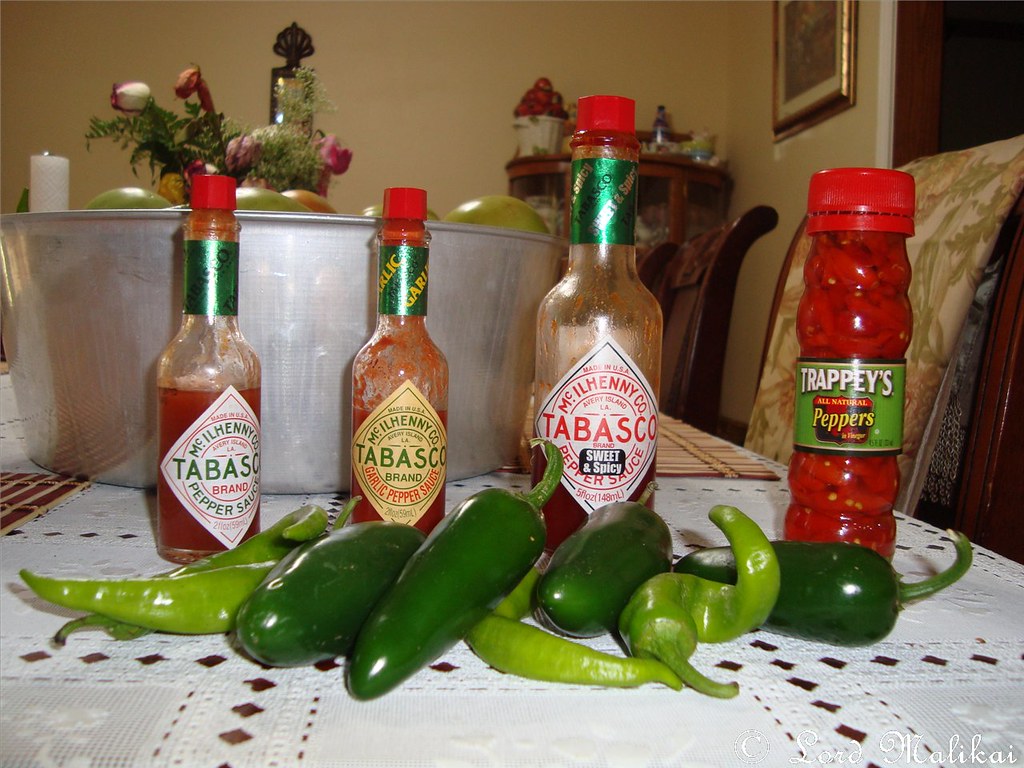The color photograph, captured indoors in landscape mode, showcases a vibrant display of various peppers and hot sauces on a table adorned with a white eyelet tablecloth and woven place mats. In the foreground, a collection of jalapeno peppers is arranged, featuring a mix of smooth, shiny dark green peppers with blunt ends, and thinner, lighter green ones, including a uniquely curly pepper. Behind them, there are three partially filled bottles of Tabasco sauce, each with distinct labels indicating different flavors: Original Tabasco, Garlic Pepper Sauce, and Sweet & Spicy Pepper Sauce. To the right of these bottles, there's a jar labeled "Trapeze All Natural Peppers," which contains sliced red peppers that resemble pimentos. The background reveals a large silver tub filled with what appear to be green apples, set against a white and yellow wall, with a framed picture hanging on the right. Additionally, a white bucket filled with unidentified red balls sits on the left, adding more color to the scene. Notably, a small inscription at the bottom right reads "Copyrighted Lord Malachi."